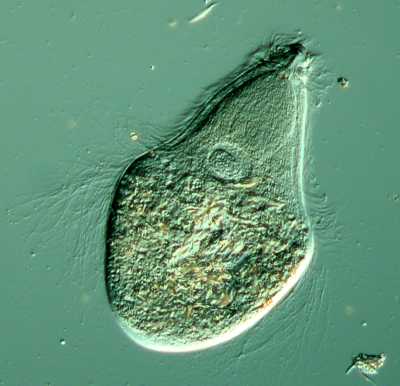This detailed close-up image, likely taken under a microscope, features a pear-shaped object that appears to be some kind of microbe, possibly a bacteria or virus. The image is predominantly green with hints of yellow. The background, a solid green square, contrasts with the textured foreground object. This central figure, rough at its base and smoother toward the top, also exhibits a circular depression around the middle. There is no identifying information provided in the image such as the type or name of the microbe, magnification level, location, or photographer details, making it more challenging to ascertain its exact nature. The object almost appears to have a stem-like structure towards the top right, adding to its distinctive pear-like appearance.